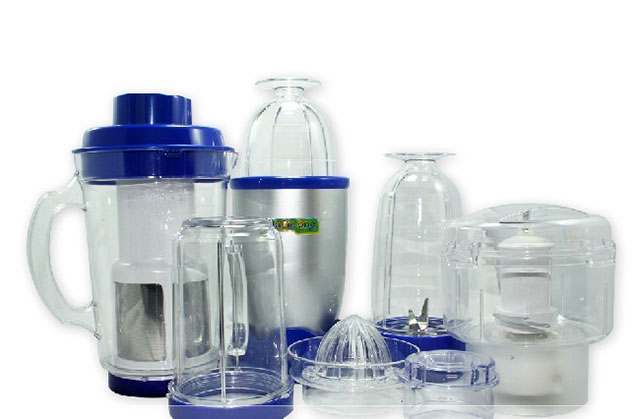This digital photograph features a detailed advertisement set against a stark white background, showcasing an array of kitchenware products primarily designed for blending and mixing. On the far left, there's a transparent pitcher with a distinctive blue base that gradually tapers as it reaches the top. In front of it sits an upside-down clear cup with a rounded blue opening at its base. Central to the image is a sleek blender that resembles a Nutribullet but appears to be of a different brand with a dark blue base, a stainless steel body, and a blue top. The blender features a yellow logo adorned with black text, though the text is not clearly legible. Adjacent to the blender, there's a manual citrus juicer designed for extracting juice from fruits like oranges and lemons, adding to the theme of health-focused kitchen gadgets. To the right, the arrangement includes another clear container with a prominent blue base, visible metal blades inside for blending, and a large clear pitcher that also seems intended for mixing or juicing tasks. These products collectively suggest a focus on smoothie preparation and other culinary tasks requiring the combination of multiple ingredients.